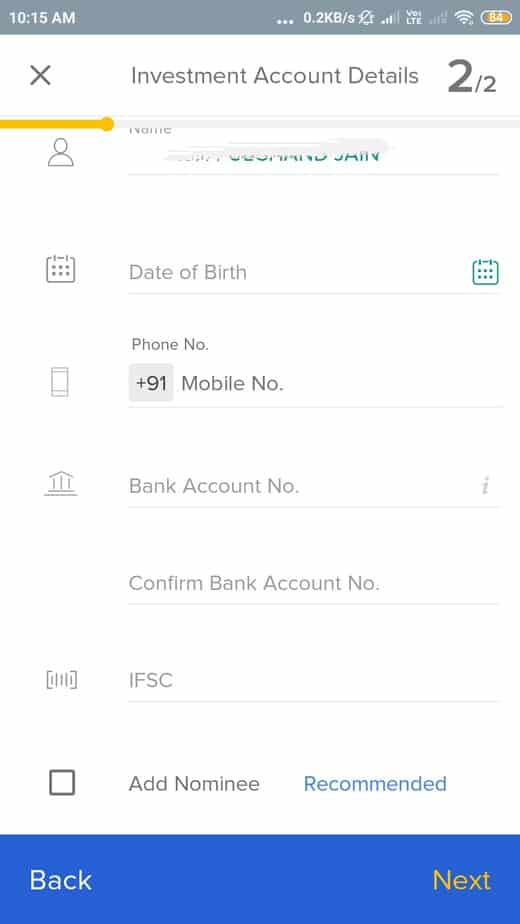The screenshot depicts page 2 of 2 of an "Investment Account Details" form. The form is primarily designed to capture personal and banking information required for creating an investment account. Key details are as follows:

- **Title and Navigation:** The form is titled "Investment Account Details," and this is the second page of a two-page form. A back button is visible on the left for returning to the previous page, while a "Next" button with a yellow color on a blue background is available on the right to proceed further.
  
- **User Section:** The user's name field is blurred out. The form includes a "Date of Birth" field with a calendar icon for easy date selection.
  
- **Contact Information:** The "Mobile Number" field shows a country code of "+91," but the actual number is not entered.
  
- **Banking Details:** The fields for entering "Bank Account" and "Confirm Bank Account" are both blank. Similarly, the "IFSC Code" field, required for bank identification, is also empty.
  
- **Nominee Information:** There is an "Add Nominee" checkbox, recommended by the form, but it is currently unchecked.

- **Status and Progress Indicators:** The top bar of the form indicates the current time (10:15), connectivity status, and battery status. A yellow progress bar below the top bar shows the completion status of the form.

- **Design and Interface:** The user interface is clean and user-friendly, featuring clearly navigable pages.

Overall, the form is well-designed to facilitate easy entry and review of investment account details, despite some fields remaining unfilled in this screenshot.